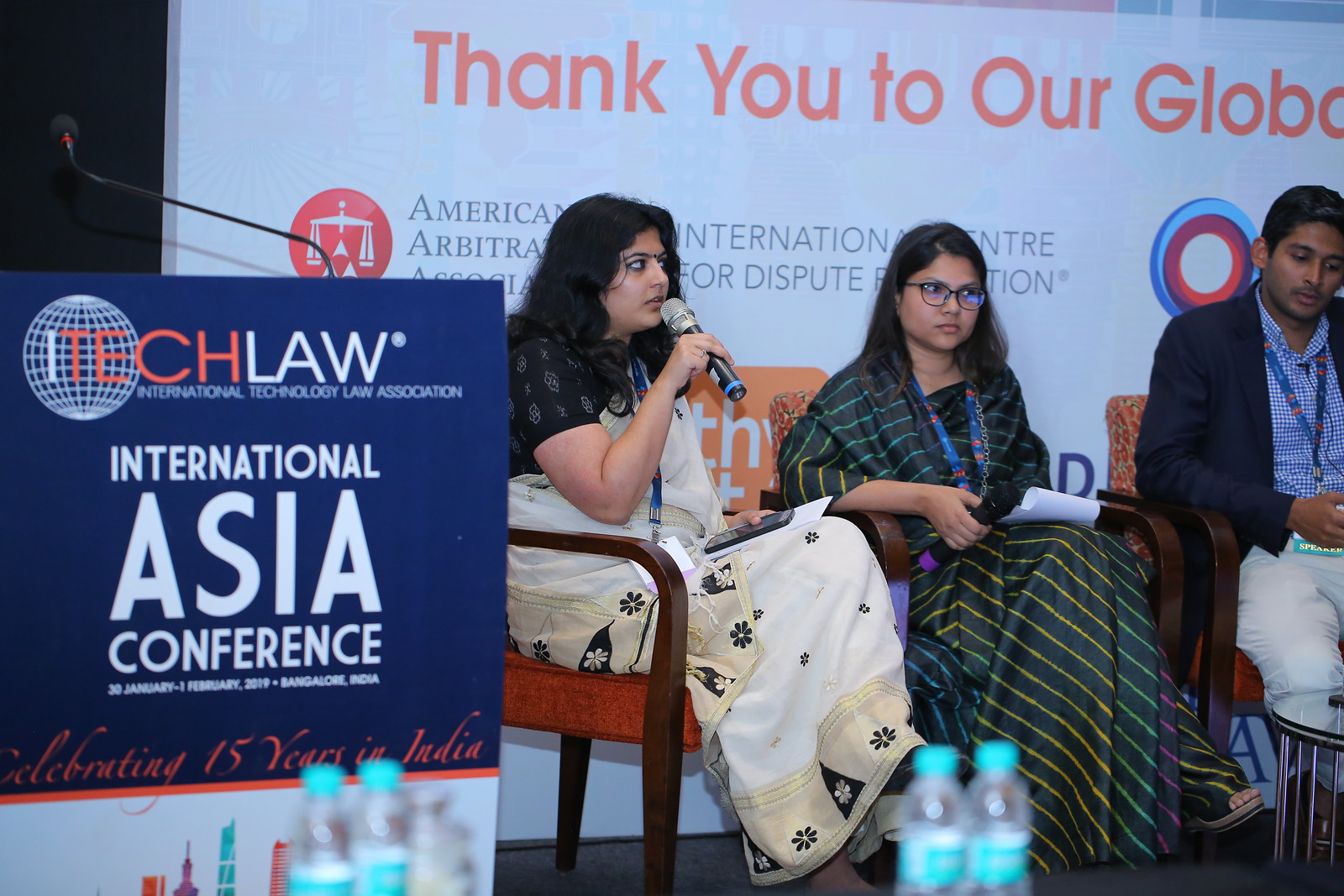This photograph captures a speaking panel at the ITEC Law International Asia Conference, celebrating 50 years in India. The event is held on an indoor stage, where three individuals are seated in orange fabric chairs. On the left, a woman with long black hair is speaking into a microphone; she is wearing a cream-colored sari paired with a black blouse, and she holds a cell phone and a document. Next to her, another woman in a flowing traditional Indian outfit and wearing glasses sits attentively. To her right, a man dressed in a jacket, blue shirt, and white pants completes the panel. All three appear to be of Indian descent and are holding notepads. Behind them, a large white banner is partially visible with the text, "Thank you to our global," along with a logo featuring a red circle with white scales of justice. To the left of the stage stands a podium inscribed with "ITEC Law International Asia Conference," including additional details like "celebrating 50 years in India." In the foreground, four water bottles with blue labels are slightly blurred, indicating the focus on the panelists.